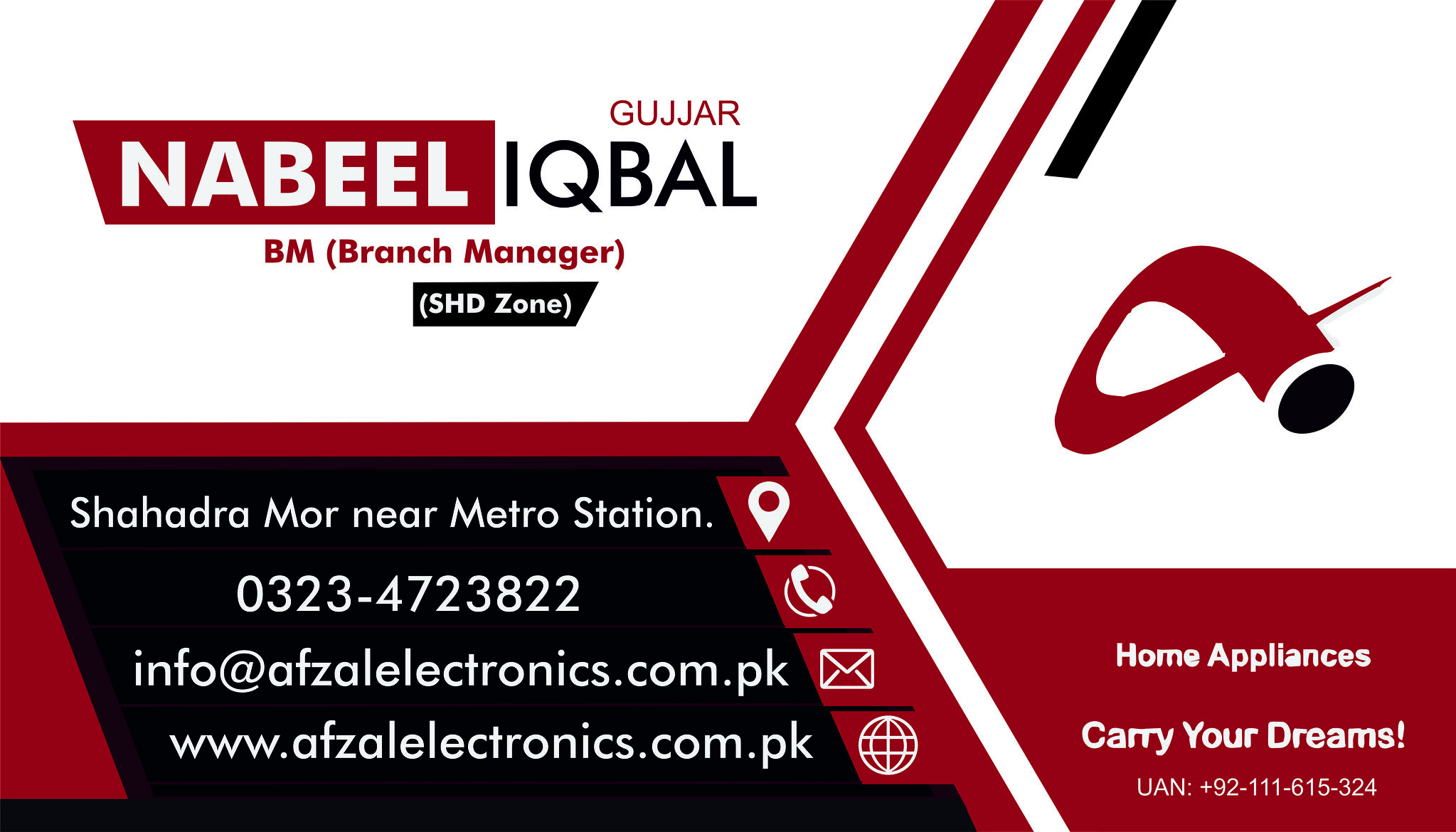This image appears to be an advertisement or business card predominantly colored in red, white, and black. On the left side, the card features the name "Nabil Iqbal Gujar," identified as the BM (Branch Manager) of the SHD Zone. Below this, in white text on a black ribbon, it says "SHD Zone." Adjacent to these details, there are various white symbols: a GPS icon indicating the location "Shahadra Moore near Metro Station", a telephone icon next to the number "0323-4723822", an envelope icon next to the email "info@afsaelectronics.com.pk", and a globe icon reiterating the URL "afsaelectronics.com.pk". Towards the center-right, there's a red logo resembling half of an infinity symbol and a black circle. Below the logo, in white text on a red background, it reads "Home Appliances, Carry Your Dreams! UAN," followed by the contact number.